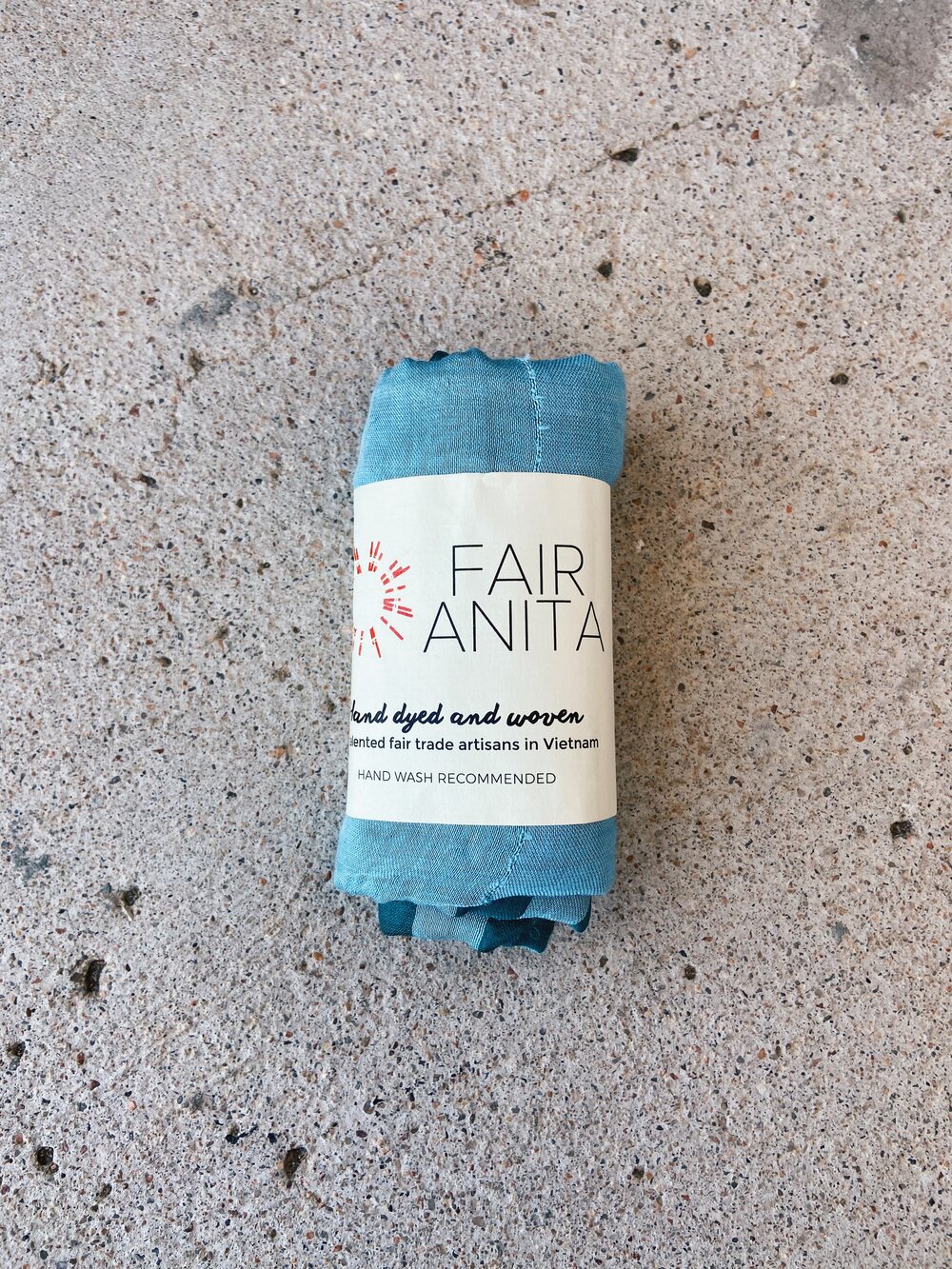This is a detailed color photograph taken outdoors featuring a blue garment, folded neatly, with a large label prominently displayed. The garment, which exhibits shades of blue, including darker blue hues, is placed on a light gray, slightly pitted concrete surface. The label, which is light in color, reads "Fair Anita" and features a small sunburst design to the left. Beneath this, the label states, "hand-dyed and woven, certified fair trade artisans in Vietnam," followed by the care instruction, "hand wash recommended." The exact type of garment is uncertain, potentially a shawl, cotton towel, or some sort of carrying case, as the left side of the label is not visible for further clarification. The item is perfectly centered in the photo, taking up about a quarter to a fifth of the frame, suggesting it is either newly bought or intended for sale.